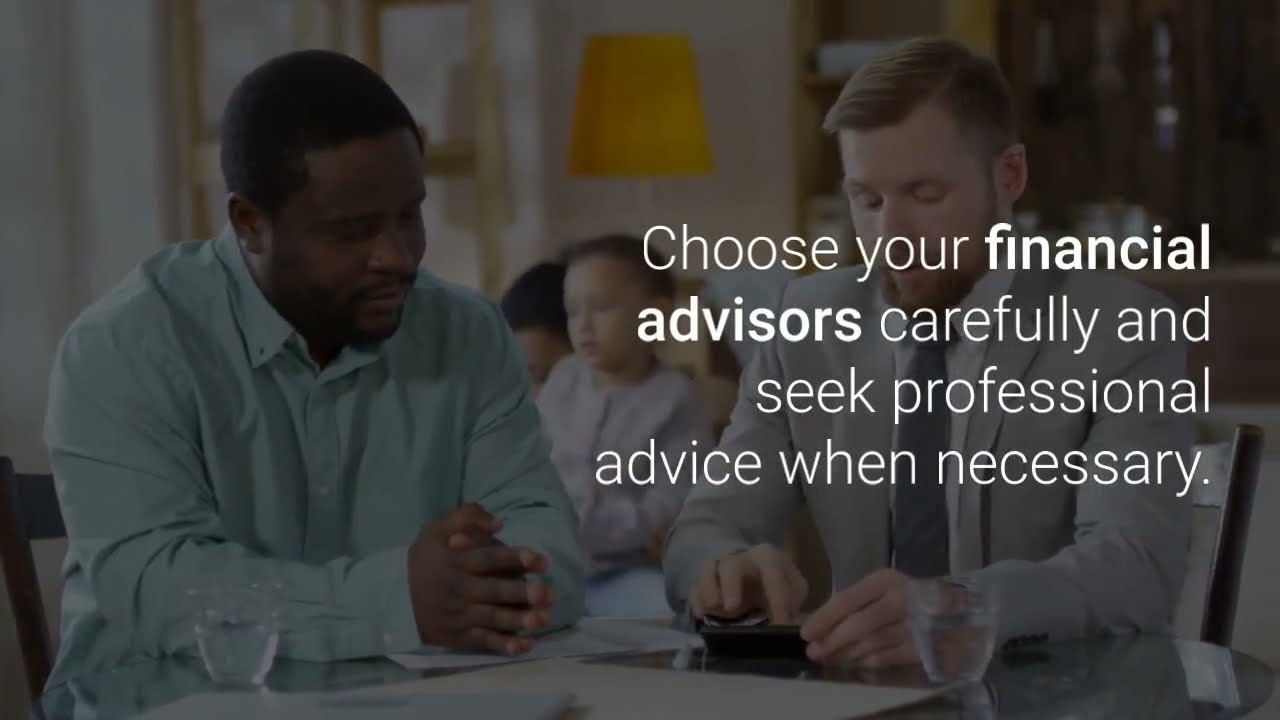This is a horizontal and rectangular advertisement featuring an image of two men in an office setting. The foreground displays a man in a light gray suit with a dark blue tie who appears to be typing on his phone. Seated next to him is an African-American man in a light blue button-down shirt, his hands clasped together on a white table, both having clear glasses of water beside them. The background is slightly darkened, featuring blurred-out figures, including a girl in a onesie and another person, suggesting a casual, lived-in environment with a white wall, yellow lampshade, and a bookcase. Overlaying the image are four horizontal rows of white text reading, "Choose your financial advisors carefully and seek professional advice when necessary," with the words "financial advisors" emphasized in bold. This detailed composition underscores the importance of prudent financial consultation.